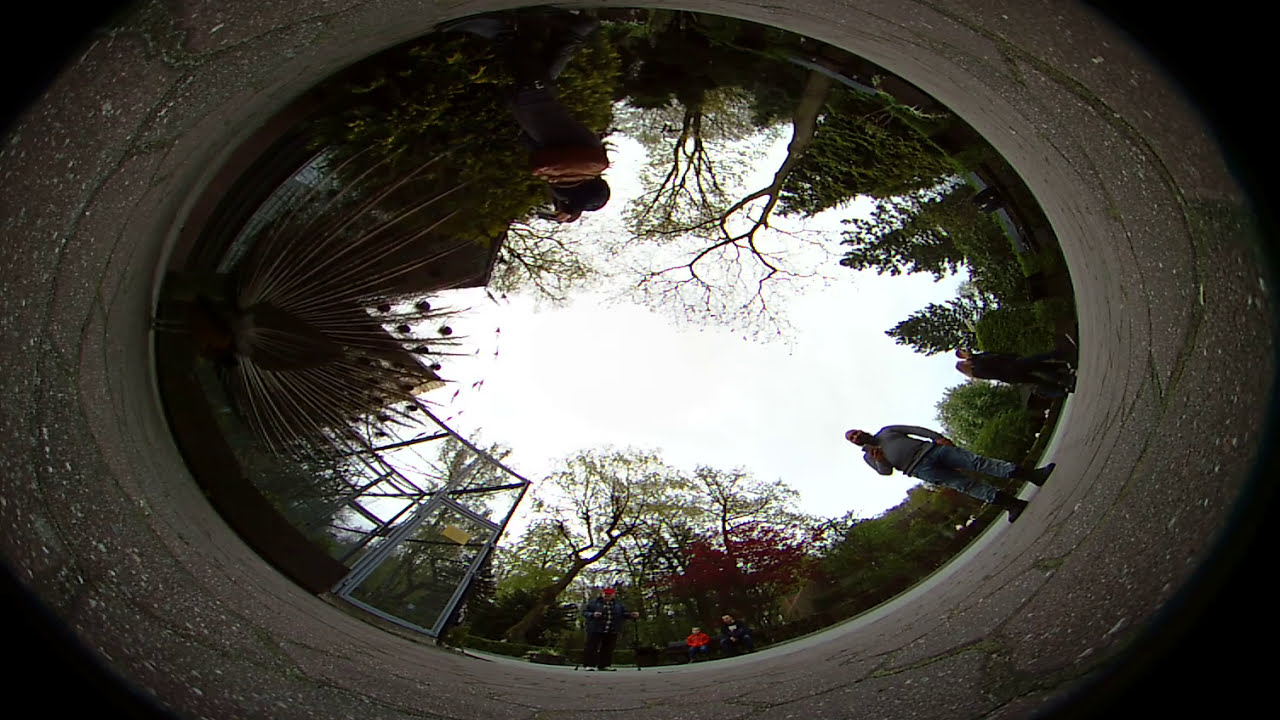The image depicts a circular, fisheye lens view of a large concrete plaza that gives the impression of a curved horizon. In the center of the image stands a person wearing a gray shirt and jeans, holding a phone in his hand. Surrounding him are other people, some walking away or towards something. The ground comprises paving stones with green lines filling the gaps. There's a steel or metal enclosure to the right side of the image. Prominently, in the top left, a peacock with its feathers fully splayed adds a unique detail. The background reveals a variety of trees, with vibrant green, red, and yellow foliage, under an overcast sky, lending a park-like, enclosed feel to the scene.